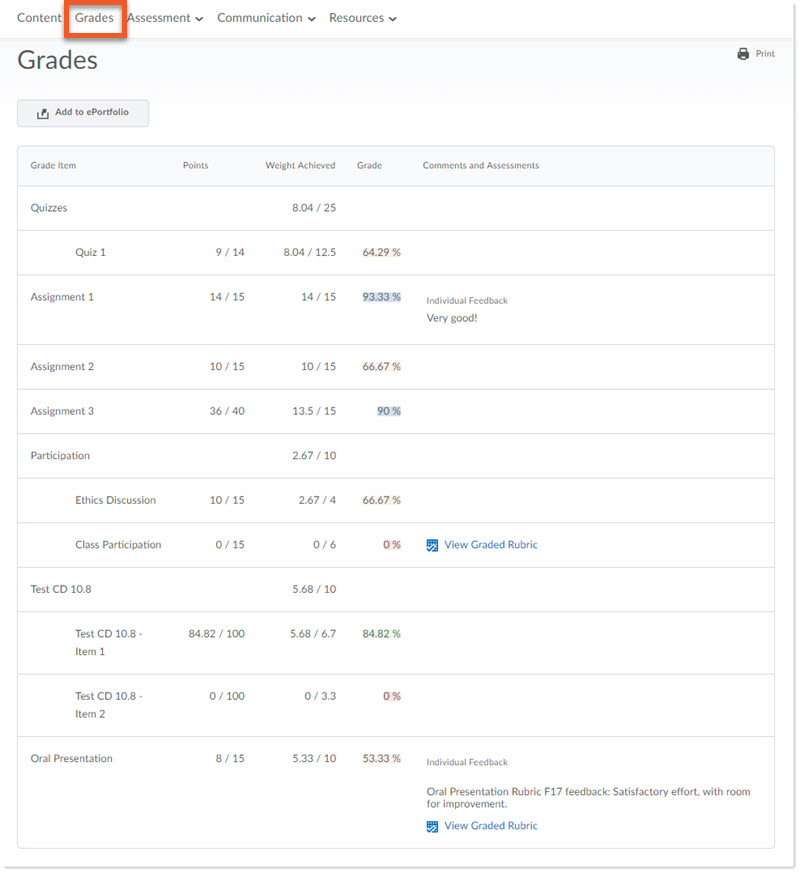In the image, we see an individual viewing an online file that displays someone's academic grades. The interface includes tabs titled: "Content," "Grades," "Assessment," "Communication," and "Resources," with the "Grades" tab prominently highlighted in a red box. The main section of the page is labeled "Grades" in large letters, followed by an option to "Add to ePortfolio."

Beneath that, a detailed table is visible, organized into columns labeled: "Grade Items," "Points," "Weight Achieved," "Grade," and "Comments and Assessments." The table comprehensively lists the grades for various assignments and quizzes.

- For "Quizzes," the weight achieved is 8.04/25. Specifically:
  - "Quiz 1" shows points of 9/14, a weight achieved of 8.04/12.5, and a grade of 64.29%.

- The first assignment, "Assignment 1," has:
  - 14/15 points,
  - 14/15 weight achieved,
  - 93.33% grade,
  - Highlighted in a purplish-blue color with a note saying "Individual Feedback: Very Good."

- "Assignment 2" scores:
  - 10/15 points,
  - 10/15 weight achieved,
  - 66.67% grade.

- "Assignment 3" displays:
  - 36/40 points,
  - 13.5/15 weight achieved,
  - 90% grade.

Following these assignments, there are subsequent sections:
- "Participation" with a weight achieved of 2.67/10.
- "Ethic Discussion," listing 10/15 points, 2.67/4 weight achieved, and a 66.67% grade.

The table continues with other categories such as "Class Participation," "Test CD," and "Oral Presentation," each detailing specific grades, points, and weights achieved for each category.